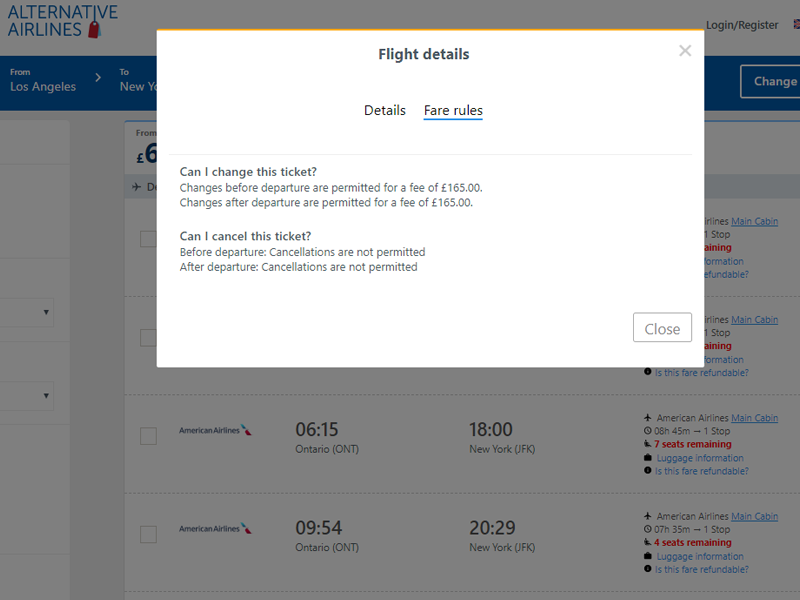The image displays a screenshot of the Alternative Airlines website. In the top left corner, the site’s logo is visible with blue text and a distinctive red icon. In the top right corner, options to "Log In" and "Register" are prominently placed. 

Central to the screenshot is a white-background pop-up with a yellow header that reads "Flight Details." Below this header, there are two sections labeled "Details" and "Fare Rules," with "Fare Rules" underlined in blue. 

The "Fare Rules" section starts with the question, "Can I change this ticket?" It indicates that changes before departure are permitted for a fee of £165. It repeats with another question, "Can I cancel this ticket before departure?" The response clarifies that cancellations are not permitted, both before and after departure.

In the top right corner of the pop-up is an "X" icon for closing, and at the bottom right is a "Close" button. 

The pop-up obstructs much of the underlying webpage, but a portion is visible, showing flight times for two departures from Ontario to New York. The first flight departs Ontario at 06:15 and arrives in New York at 18:00. The second flight leaves Ontario at 09:54 and arrives in New York at 20:29. 

On the right-hand side of the page are a few links in blue text and an indication of the number of remaining seats, highlighted in red.